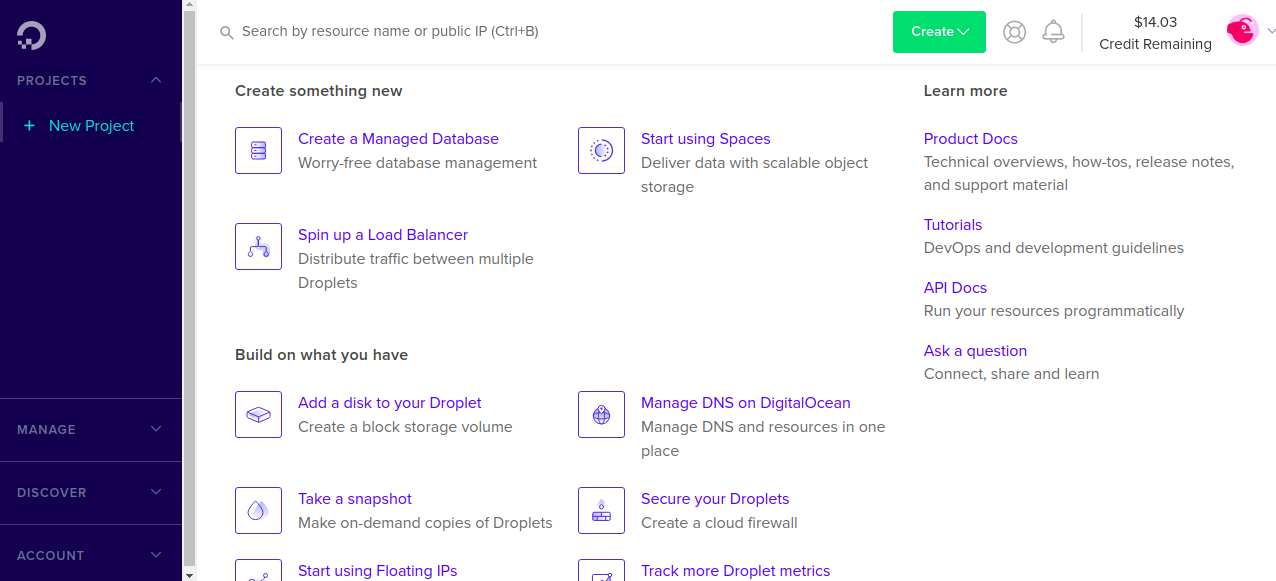**Detailed Caption:**

This screenshot displays the user interface of an unnamed service or program. The layout is divided into two primary sections. 

On the left-hand side, there is a vertical navigation pane. At the top of this pane, you can see the icon representing the program. Beneath it, there is a section titled "Projects," where users have the option to add a new project. Lower down in this pane, three distinct boxes are labeled "Manage," "Discover," and "Account." Additionally, the presence of a scrollbar indicates that there are more categories accessible by scrolling within this frame.

The right side of the image showcases the main interface of the program, capturing the expansive screen space typical of a wide computer monitor. The header at the top of this section includes several key elements: 
- A search bar prompt reading, "Search by Resource Name or Public IP"
- A "Create" button
- A few icons, one of which is unclear, and another representing an alarm
- A balance display showing "$14.03 in credits"

Directly below this header bar are various functional buttons designed for users to:
- "Create a managed database"
- "Start using Spaces"
- "Spin up a load balancer"
- "Build on what you have"

Following these primary actions, several other items are presented. On the far right of the main section are resources for further learning, which include:
- "Learn More"
- "Product Docs"
- "Tutorials"
- "API Docs"
- "Ask a Question"

The detailed elements and organized layout suggest that this interface is part of a comprehensive management or development platform, providing users with a range of functionalities and support resources.